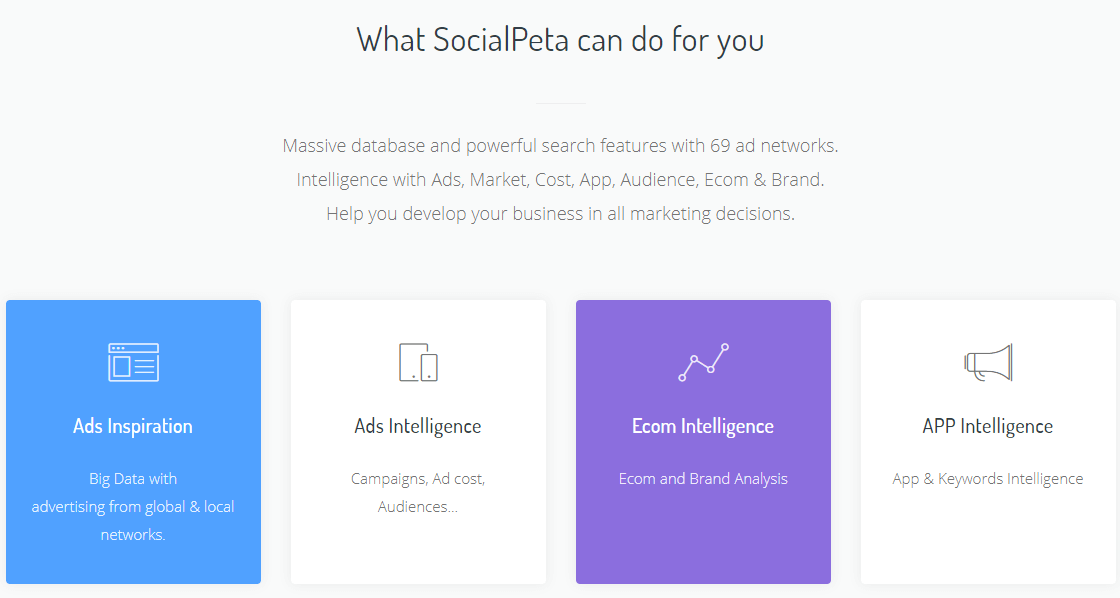This image showcases a web page, prominently featuring information about the capabilities of SocialPETA. At the top center of the image, the headline reads, "What SocialPETA Can Do For You." Directly beneath this headline, a subheading details SocialPETA's key offerings: a massive database, powerful search features spanning 69 ad networks, and tools for making informed marketing decisions, including ads, market, cost, app, audience, e-commerce, and brand data. 

Further down, the page is organized into four distinct boxes, each highlighting a different feature:

1. **Ads Inspiration** (Blue Box, White Text): This section emphasizes the extensive advertising data collected from both global and local networks.
   
2. **Ads Intelligence** (White Box, Black Text): Here, users can find insights into ad campaigns, costs, audiences, and more.

3. **E-com Intelligence** (Light Purple Box, White Text): This box focuses on e-commerce intelligence, offering analysis of e-commerce trends and brand performance.

4. **App Intelligence** (White Box, Black Text): This final section provides intelligence on app and network performance.